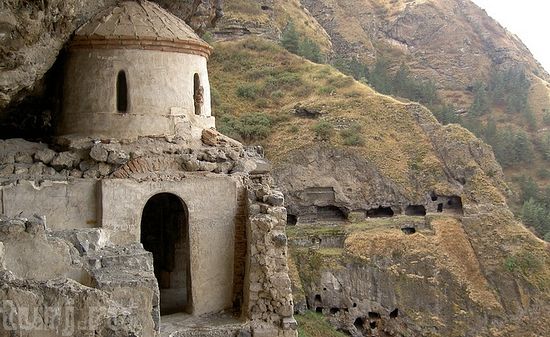This outdoor photo showcases a rugged mountainous region, likely European, characterized by a rocky hillside with sparse, low-growing vegetation and some distant trees. Dominating the left side of the image is a two-story stone building, beige in color, seemingly carved directly out of the rock of the mountain. This cement or adobe shelter features a distinctive arched doorway and two open, arched windows on the upper level. The building also has a domed roof, blending seamlessly into its rocky surroundings. The landscape is dotted with several caves, seven of which are centrally located, while a few others are dispersed lower and higher on the mountain. In the upper right-hand corner of the image, a patch of white sky is visible, underlining the isolation and natural grandeur of the scene.